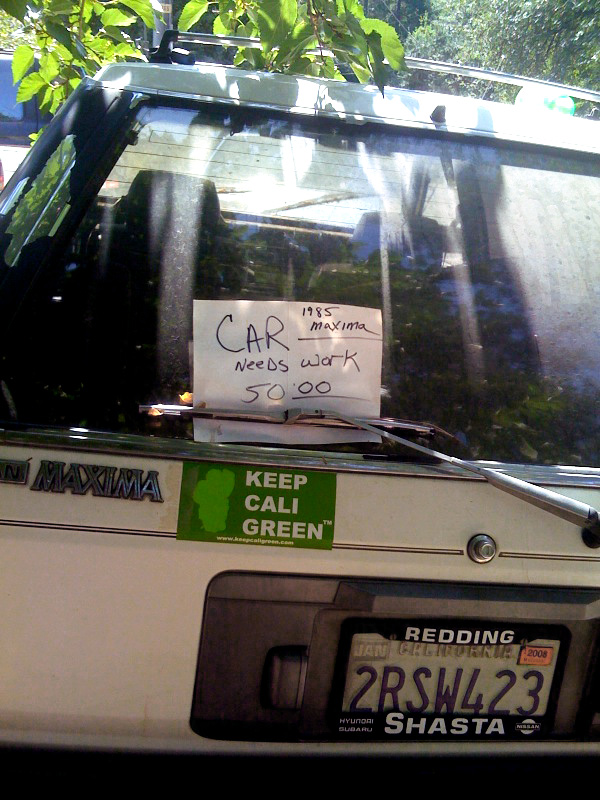This image captures a close-up view of the rear end of an old, boxy, silver station wagon, likely from the 1980s. The shot is taken outdoors under the shade of trees, providing a backdrop of leafy branches that frame the upper part of the vehicle. Prominently displayed in the center of the rear windshield, held in place by the resting back windshield wiper, is a standard-sized piece of white paper with handwritten black text. The sign reads "CAR 1985 Maxima needs work $50," with "1985 Maxima" positioned in the upper right corner and "$50" underlined, possibly indicating cents. Below the sign, on the left side of the hatchback, the vehicle's branding indicates "Maxima." Adjacent to this, a green bumper sticker declares "Keep Cali Green" in white letters. The car's license plate, surrounded by a border that reads "Redding Shasta Hyundai Subaru," displays the number "2RSW423" with registration details showing January 2008 for California.